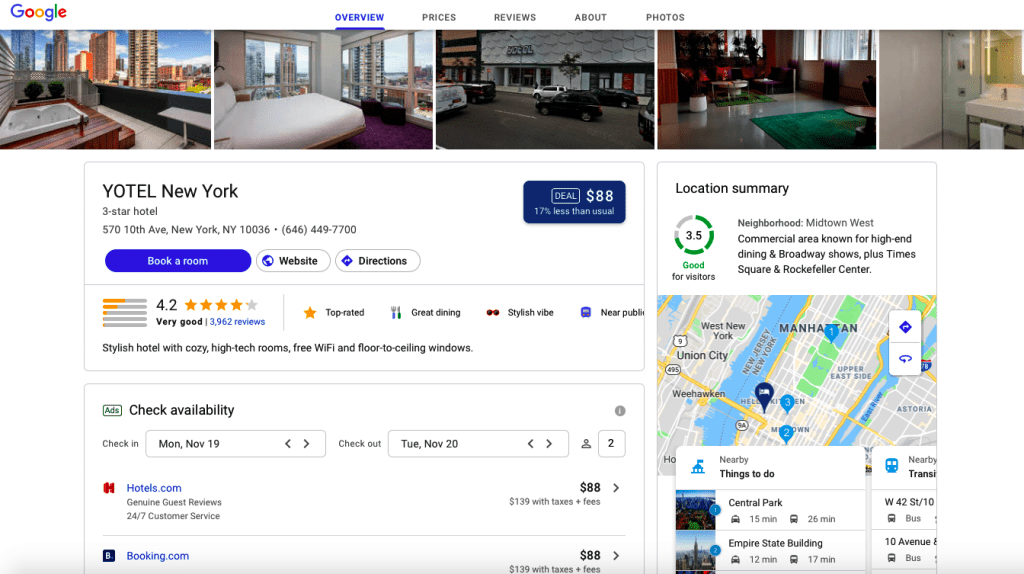The image showcases a detailed webpage for Yotel, a three-star hotel located in New York, New York. At the top left corner, the page is branded with the Google logo. A horizontal menu bar follows, presenting options labeled "Overview," "Prices," "Reviews," "About," and "Photos," with the "Overview" tab highlighted in bright blue, while the other options are in gray font.

Directly beneath the menu options, there is a horizontal gallery of five images depicting various rooms, buildings, and scenes possibly related to the hotel's interior and surroundings. Notably, the fifth image is slightly smaller than the others.

The main body of the page features the hotel's name, "Yotel," prominently displayed in bold, black, all-capital letters. Beneath "Yotel," "New York" is shown with just the "N" and "Y" capitalized. Subsequent to the hotel name, detailed information is listed: "Three Star Hotel," the address "570 10th Avenue, New York, New York, 10036," and a contact phone number.

To the right of this information, there's a blue horizontal rectangular box with "DEAL" written in white, uppercase letters, enclosed by a white border. Adjacent to this box, white text displays the price "$88," with a note indicating that this rate is "17% less than usual."

Below the hotel name and details, there is an option to "Book a Room" in a blue horizontal oval with white lettering, followed by a "Website" button and a "Directions" button, both set on a white background with black text.

Underneath, the hotel's rating is presented: a 4.2 out of 5 depicted with four gold-colored stars and captioned as "Very Good." Accompanying this rating are specific notations such as "Top-rated," "Great dining" marked with a fork and knife icon, "Stylish vibe," and "New profile."

Further down, there is a "Check Availability" section, and to the right of it, a "Location Summary" that highlights a 3.5 rating within a circular indicator partially bordered in green. The section specifies "Good" in green text and describes the neighborhood as "Midtown West," a commercial area noted for high-end dining, Broadway shows, Times Square, and Rockefeller Center. Below this summary, a map is displayed for additional context.